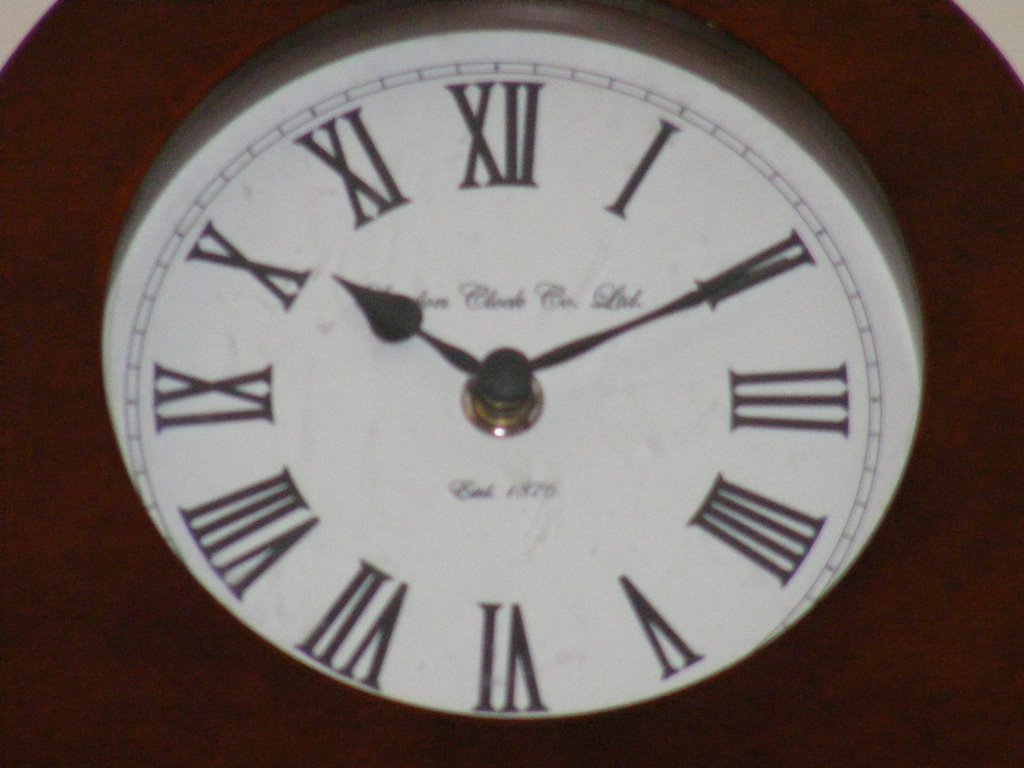This color photo features an up-close view of a clock face, predominantly displaying the central and lower parts. The clock's case is made of dark brown wood, curved along the sides, with the top part of the clock cut out of the frame. The clock face itself is white, adorned with black Roman numerals. Surrounding the center, they are correctly positioned as follows: XII at 12 o'clock, I at 1 o'clock, II at 2 o'clock, III at 3 o'clock, IV at 4 o'clock, V at 5 o'clock, VI at 6 o'clock, VII at 7 o'clock, VIII at 8 o'clock, IX at 9 o'clock, X at 10 o'clock, and XI at 11 o'clock. The clock is set to 10:10, with the longer minute hand pointing at the 2 and the shorter, thicker hour hand just above the 10.

In the center of the clock, partially obscured by the hands, is some writing that reads, "Clock Company Limited. Established 1875," although parts of it are blurred and out of focus.